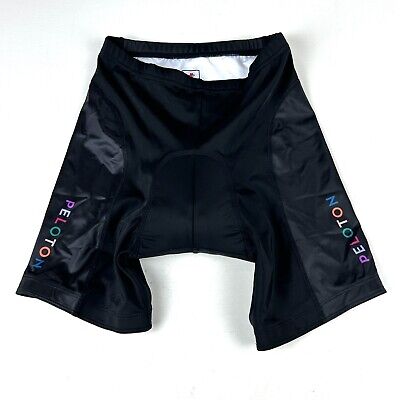This image depicts a pair of black athletic shorts, likely designed for biking or running, displayed flat on a white surface, with no additional background context. The shorts are made from a shiny, breathable fabric with an elastic waistband, and feature a white interior lining. Each leg of the shorts displays the word "PELOTON" vertically in a multi-colored font. On the right leg, the letters start from the hip and read downward: P (pink), E (white), L (pink), O (light blue), T (white), O (light pink), and N (slightly darker pink or light red). On the left leg, the letters start from the bottom and read upward, arranged in reverse order: N (light pink), O (light pink), T (white), O (light blue), L (pink), E (white), and P (pink). The side panels of the shorts are made from a different material than the main body, emphasizing the air-permeable design intended to enhance comfort and sweat absorption. The overall appearance suggests a spandex-like feel that likely allows for a snug, supportive fit.